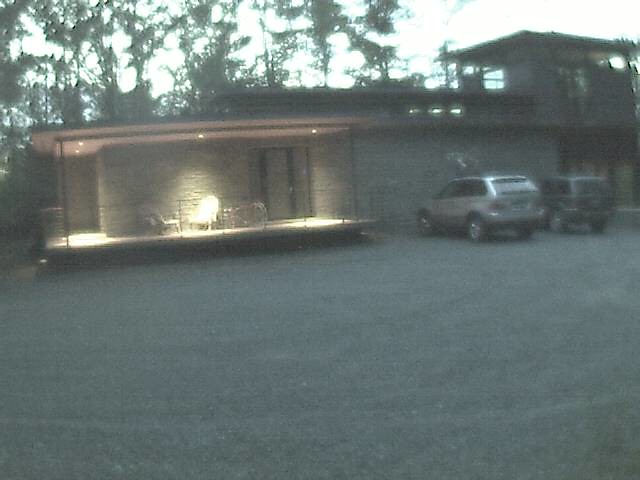The image captures a gravel driveway leading up to a building that may have once been a school but now appears to be a residential property. On the left side of the scene, there is a deck that features brick construction and is adorned with lighting. The deck also houses a couple of chairs and has a single sliding door that suggests it's used for outdoor lounging. In the far background, a dense array of trees hints at the location being a large or rural property. On the right side, two vehicles are parked: a black Road Ranger and a silver Kia. The building itself boasts architectural elements reminiscent of a school, including double doors, an above watch area, and a smaller storage section.